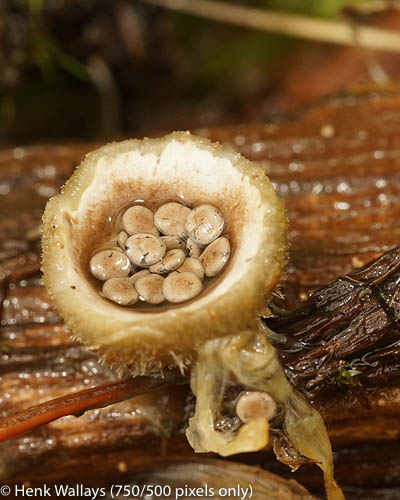This detailed close-up photograph captures an enigmatic organic object lying against a glistening, tree bark-like surface. This object resembles an open, flower-shaped, yellow-brown mushroom, possibly a peculiar fungus, featuring a collection of small, round, brown seeds nestled in its white interior, giving it a textured, almost furry exterior. A sticky, gooey substance appears to be exuding from its lower right side. The background of the image displays blurred green vegetation and sap-coated brown wood, adding to the natural setting. In the bottom left-hand corner, white text indicates the copyright symbol "©" followed by "Henk Wallays (750/500 pixels only)."